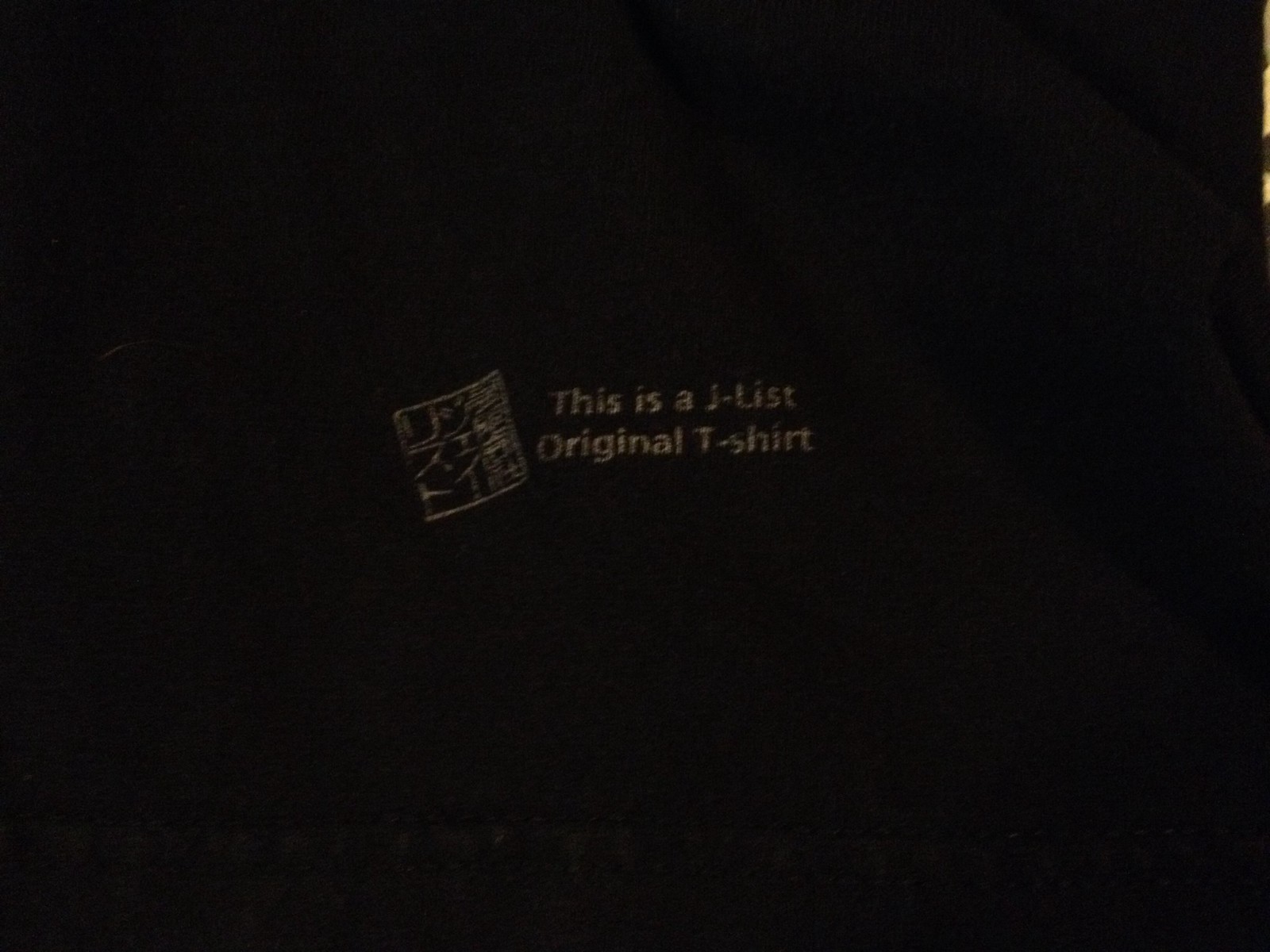The photograph showcases a section of black fabric with light yellow text printed on it. In the top right corner, the cloth has noticeable creases. The text, which appears slightly faded reminiscent of an aged t-shirt, reads "This is a J-List original T-shirt." Adjacent to this text on the left, there is a square outline containing Japanese characters, giving the impression of a traditional Japanese 'chop' or seal. Although the square is slightly angled, it is not at a 45-degree angle. Both the text and the square design are rendered in a dark gold hue, suggesting they might be made from heat transfer vinyl.